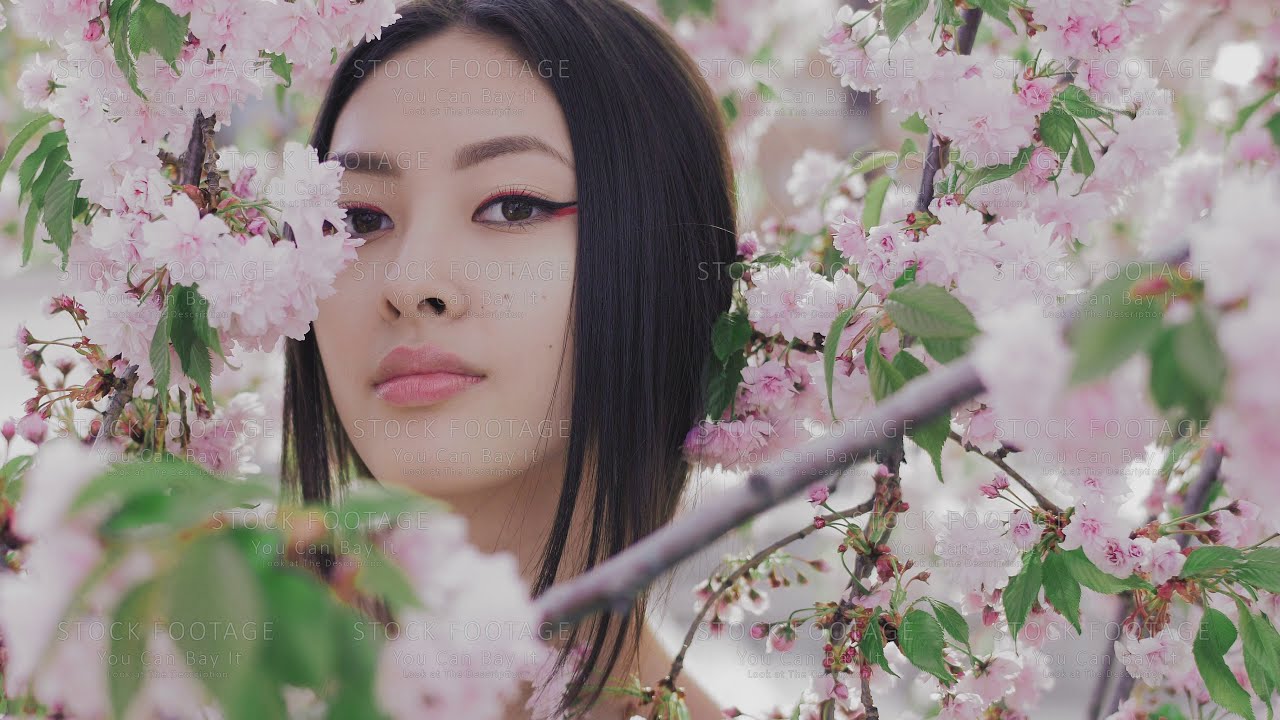The image features an Asian woman with a medium to short bob cut of straight black hair, accentuated with tufts extending down the sides of her face. She stands amidst an array of light pink to purple flowers, partially behind some blooms, creating a lush, vibrant backdrop of blossoms interspersed with green leaves and branches. She gazes directly at the camera, her face adorned with mascara enhancing her brown eyes, pink lipstick accentuating her lips, and a subtle touch of red eyeshadow adding a hint of color around her eyes. The photograph is overlaid with a faint gray watermark that reads "stock footage," along with smaller, indistinguishable text beneath it.